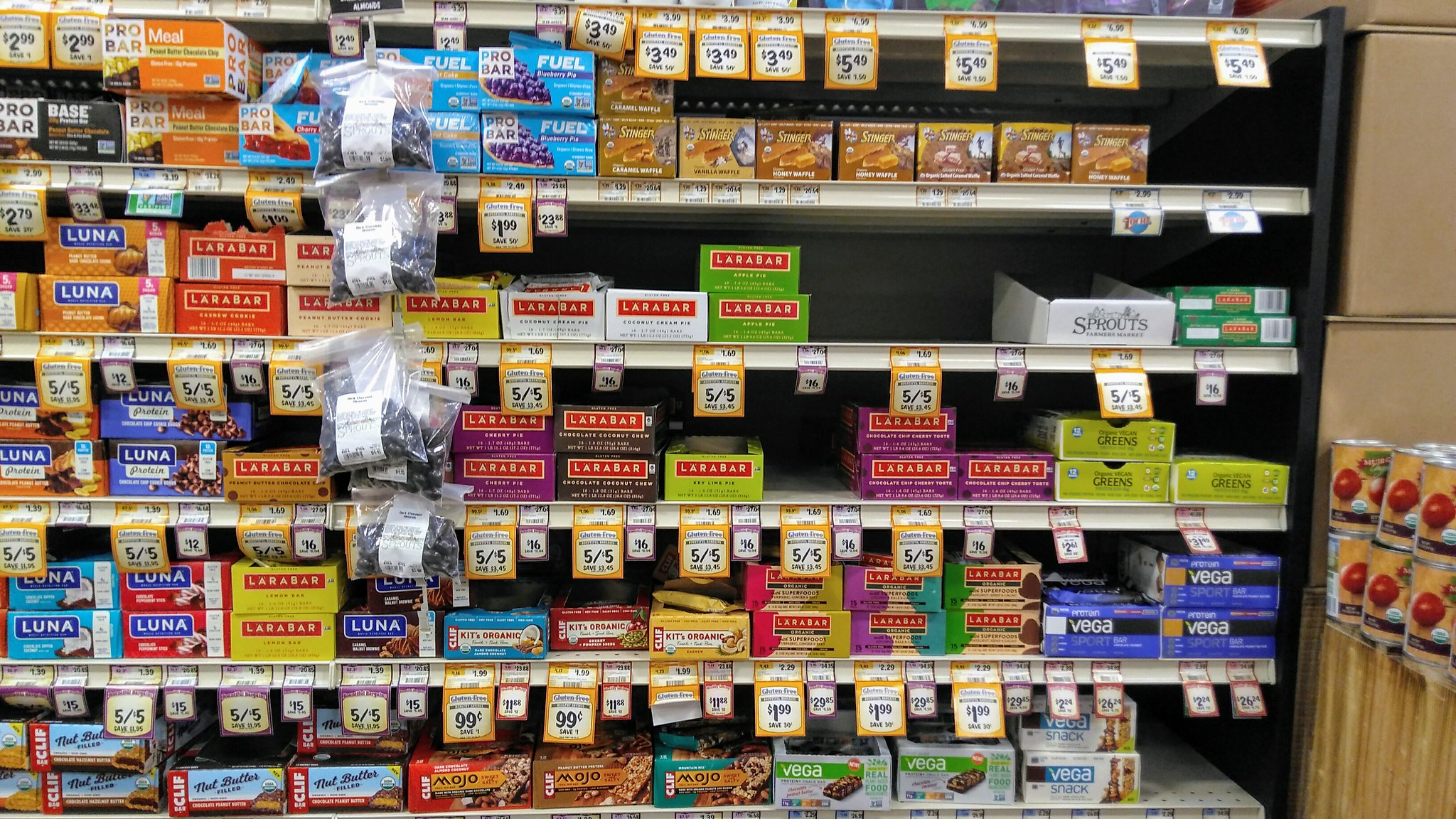In this color photograph taken inside a grocery store, five to six shelves display a variety of health products, predominantly Luna and Voob bars. The shelves are lined with small, colorful boxes, including combinations like orange with blue, red with white, yellow with red, and others. On the far right, there are six cans stacked two high, possibly featuring tomatoes on them, with some cardboard boxes overhead. The shelf fronts are silver, and the ends are black, with numerous black, yellow, and white price tags. Additionally, a small white paper labeled "Sprouts" suggests this could be a Sprouts store. To the left, items are densely stocked, while the right side appears more sparse. Hanging items in clear plastic bags are visible but not clearly identifiable.